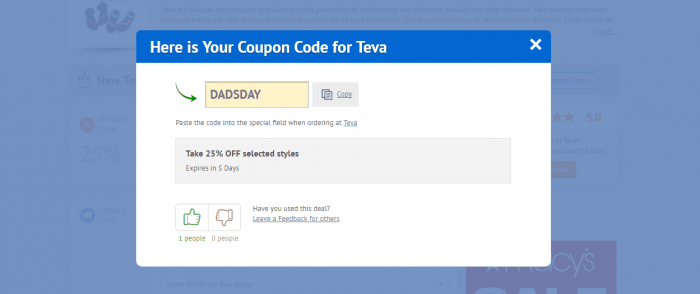The image appears to be a screenshot of a computer screen featuring two overlapping layers. The bottom layer, which has a bluish-gray overlay, makes any text or visuals beneath it difficult to discern. Overlaid on this is a prominent white rectangle with a blue header containing the text "Here is your coupon code for Teva" and an 'X' in the upper right corner.

Inside this rectangle, there is a green arrow pointing towards a text box filled with "DAD'S DAY" in all capital letters. Below this, an instruction reads, "Paste the code into the special field when ordering at Teva."

Further down within the white rectangle is another gray-background rectangle proclaiming "Take 25% off selected styles. Expires in five days." Beneath this are icons for thumbs up and thumbs down, with "1 person" indicated under the thumbs up and "0 people" under the thumbs down. This section invites users to leave feedback with the prompt "Have you used this deal? Leave feedback for others."

The partially visible underlying image has the recognizable Macy's logo at the bottom, partly covered by the white rectangle, making it difficult to read the full content except for the fragment "Sal" following Macy's. Due to the overlay and positioning of the top rectangle, further details on the bottom image remain obscure.